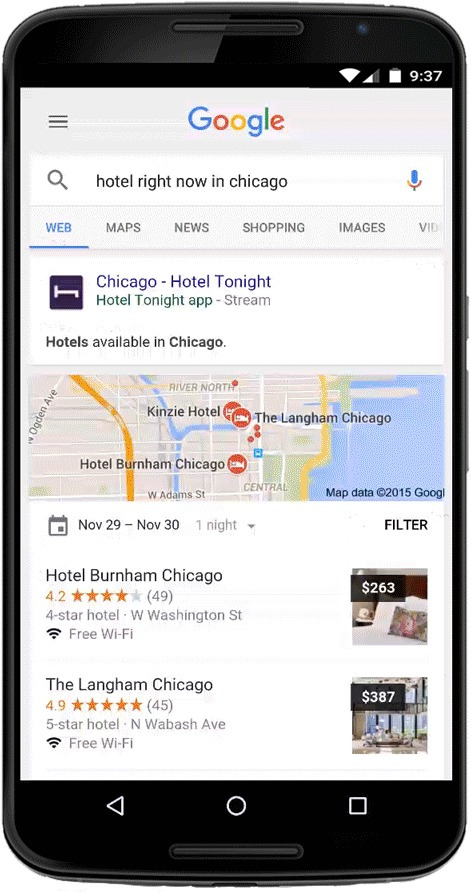This image, captured on a cell phone, showcases a Google search page. The familiar multicolored "Google" logo sits prominently at the top of the screen. The phone appears mostly black, with the search area displaying a predominantly white background, tinged with a slight tan hue. The search query entered reads "hotel right now in Chicago," and the results are displayed under the "Web" tab, though options for "Maps," "News," "Shopping," "Images," and more are available.

Several search results are visible, including "Chicago hotel tonight," "Hotel Tonight app," "Hotels available in Chicago," and more. On a partial map of Chicago, red circles with white bed icons indicate hotel locations. You can also discern some of the city's roads and the lake's water body near Chicago. The search specifies dates from November 29th to November 30th for a one-night stay, with visible hotel options such as "Hotel Birmingham Chicago" and "Langham Chicago."